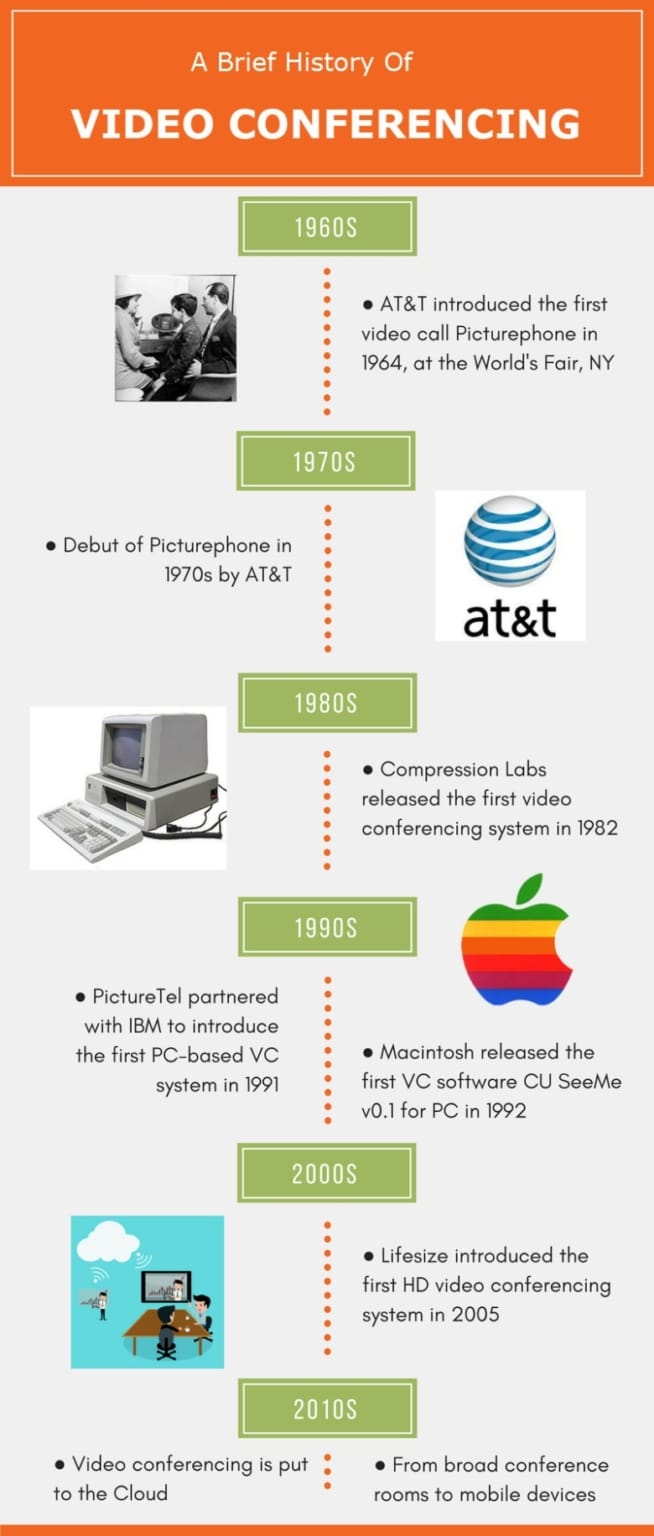The infographic titled "A Brief History of Video Conferencing" presents a chronological overview of the major milestones in video conferencing technology. At the top of the image, an orange bar with white text introduces the subject. Just above it, in a green box with white text, the timeline begins with the 1960s. 

In the 1960s section, a black-and-white photo features two women and a man using AT&T's picture phone, introduced in 1964 at the World's Fair in New York. The timeline proceeds to the 1970s, marked by another green box stating "1970s," accompanied by the AT&T logo. It notes the debut of the picture phone by AT&T during this decade. 

Moving into the 1980s, the infographic highlights Compression Labs' release of the first video conferencing system in 1982, alongside an image of an early computer setup. The 1990s segment features two key developments: PictureTel's collaboration with IBM in 1991 to introduce the first PC-based video conferencing system, and Macintosh's release of the first video conferencing software, "See You, See Me" version 0.1 for PC in 1992. This section includes images of the respective logos and iconic devices of the time.

The 2000s section shows an illustration of a video conference call, noting that LifeSize introduced the first HD video conferencing system in 2005. Finally, the 2010s section describes the shift of video conferencing to the cloud and mentions the expansion from broad conference rooms to mobile devices.

Throughout the graphic, the decades are marked with green rectangles with white text, while the rest of the layout uses black text against a gray background, providing a clear and structured journey through the history of video conferencing technology.